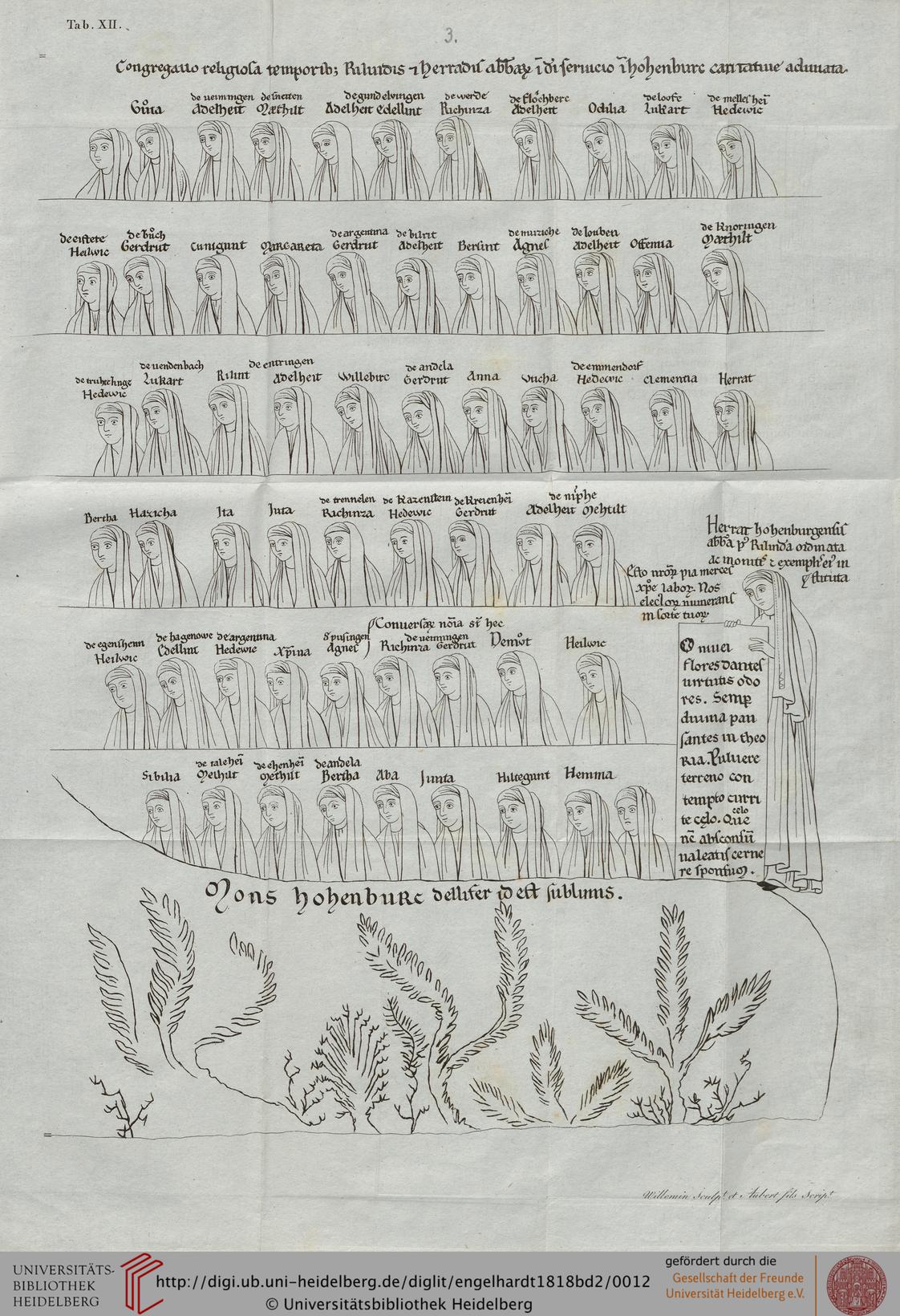This is a detailed, historical illustration featuring a series of six rows with multiple black and white drawings of women from the chest upwards, each wearing a headscarf. These women appear to have names or titles written above them in what could be Latin or German. The top of the image contains some explanatory text, likely in Latin or German, suggesting its educational or reference purpose. On the right side of the image, there is a full-length drawing of a woman dressed similarly in robes and a headscarf, holding a banner with additional Latin text. At the bottom of the illustration, there is more Latin text accompanied by drawings of various plants. The image seems to originate from a historical archive, possibly from the Universitas Bibliotheca Heidelberg, as indicated by a note or web address at the very bottom.